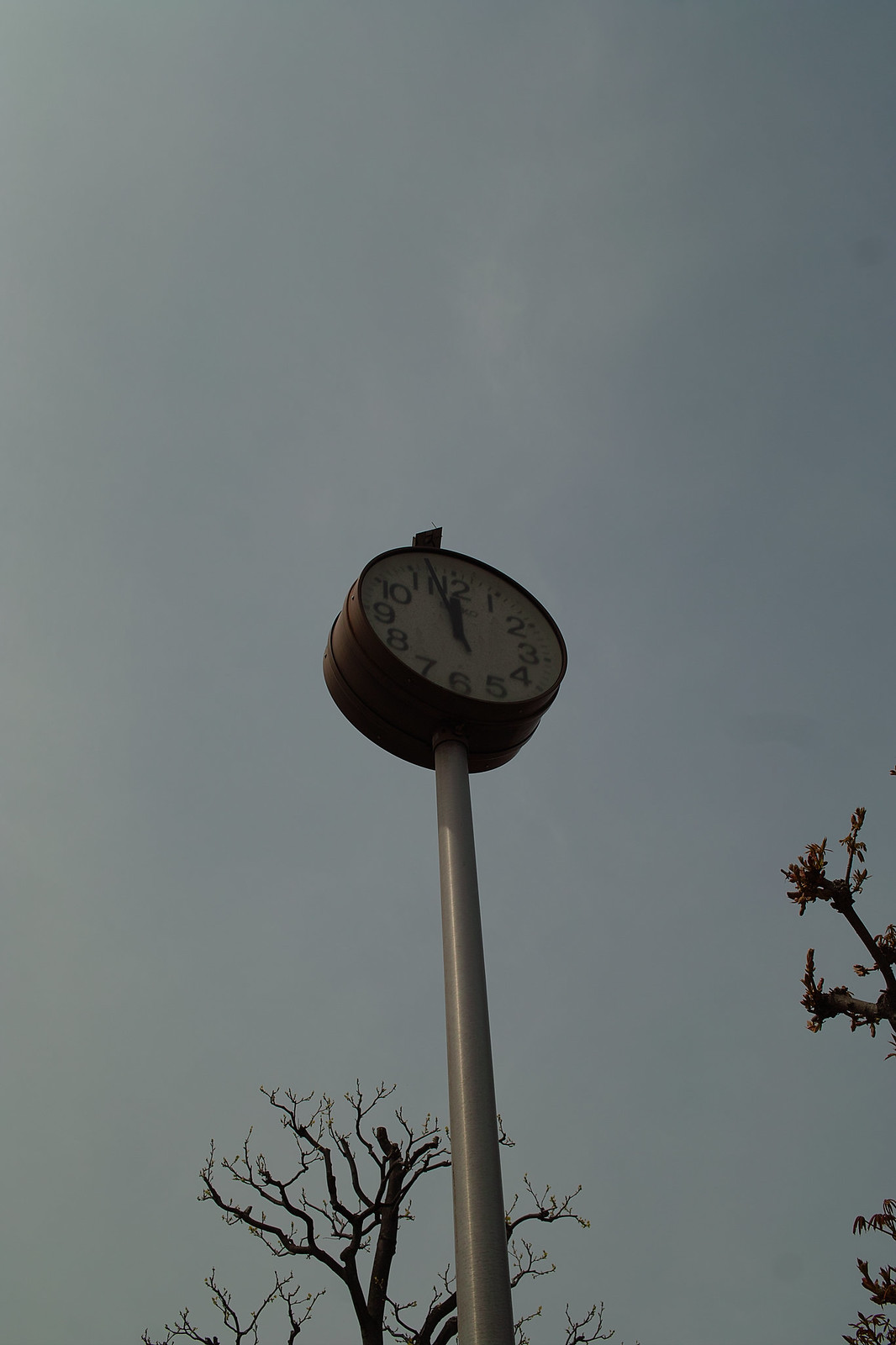The image captures an upward view from the ground, focusing on a tall pole that extends into the sky. At the very top of the pole, there is a round clock embedded within what resembles the rim of a car wheel. The pole appears to pass through the center of this rim, supporting the clock. The clock face is white, with clearly visible black numerals. Both the minute and hour hands are nearing 12 o'clock. The background displays a grayish sky, and a few barren tree branches extend upwards from the bottom of the image. On the right side, additional branches, possibly budding, are also visible. The scene prominently features the pole with the wheel-like clock against a muted, overcast sky.